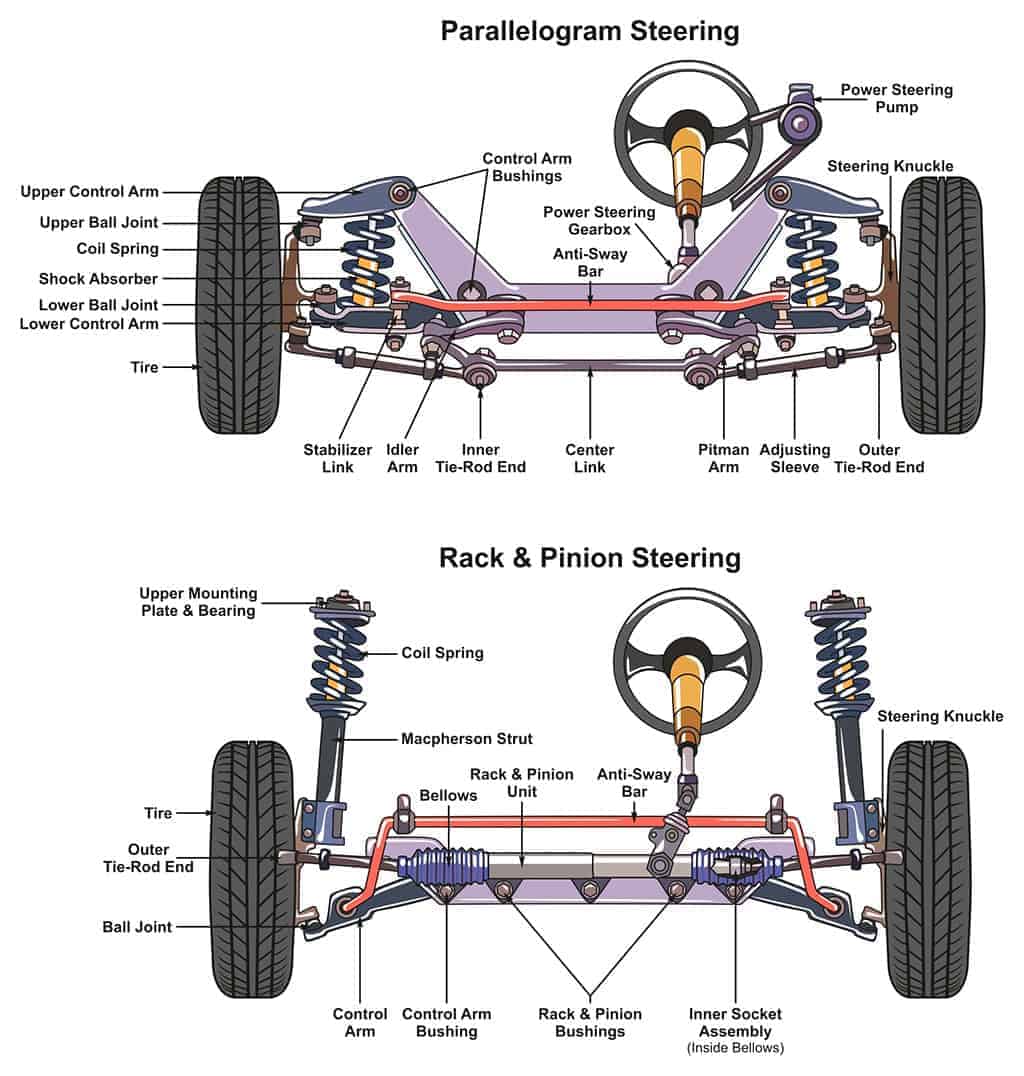This image is a detailed color illustration featuring two diagrams of car interiors, comparing different types of steering mechanisms. The top illustration, labeled as "parallelogram steering," provides an extensive front-to-rear x-ray view of a car's chassis. It displays numerous mechanical components, such as two gray tires, the lower ball joint, tire, shock absorber, coil spring, ball arm bushings, power steering pump, and steering knuckle. Each part is meticulously labeled with arrows pointing to the corresponding sections, making it clear and informative. A distinctive silver steering wheel with a tan base is visible on the right side of the car.

The bottom illustration, labeled "rack and pinion steering," showcases a similar x-ray view of the car's interior, with visible alterations. Notable components include the control arm, control arm bushing, rack and pinion bushings, and inner socket assembly. The suspension arms are prominently displayed with coils elevated high in the air to enhance visibility. Like the top diagram, it features multiple labels with small black sans serif font pointing directly to various parts, providing a comprehensive comparison of the two steering systems.

Both illustrations are hand-drawn, offering an accurate yet stylized depiction of the front portions of the car's chassis, allowing viewers to understand the inner workings of each steering mechanism effectively.